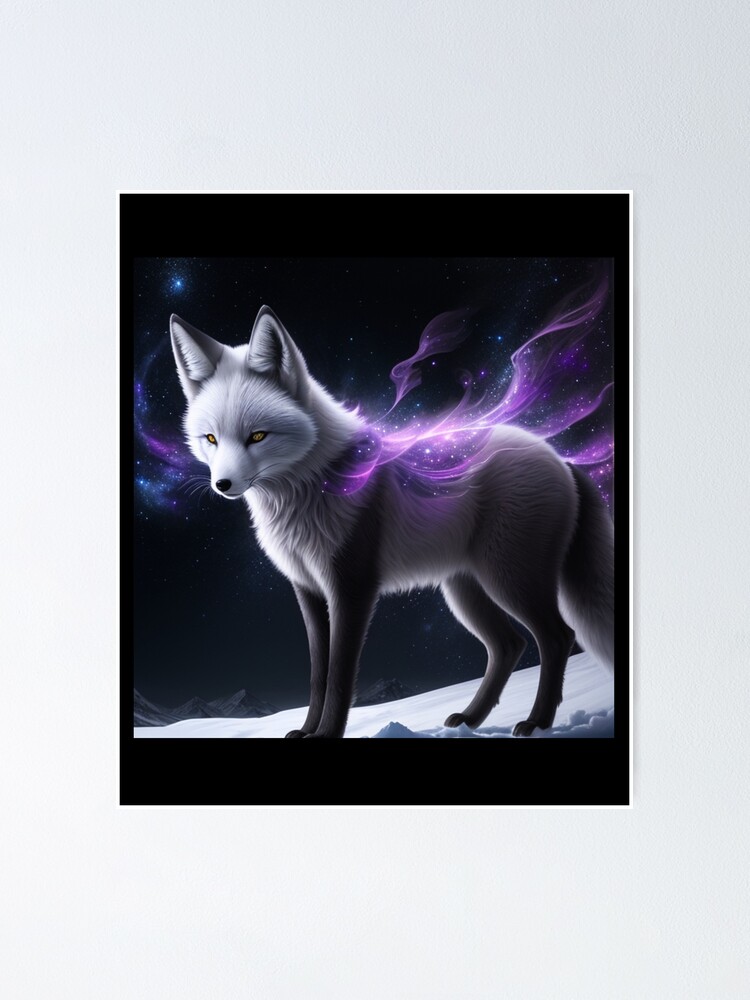This poster illustration presents a striking depiction of a wolf set against a stark black background, standing majestically in the snow. The wolf, rendered in light gray fur with dark gray accents on its ears, legs, and back, has piercing yellow eyes that gaze intently to the left. Emanating from its body are luminous, flame-like extensions in vibrant shades of fluorescent purple and blue, resembling radiating energy or ethereal wings. These colorful extensions, which include hints of stars and celestial bodies, lend the image an otherworldly, almost galactic aura reminiscent of the northern lights. The detailed portrayal, coupled with the contrasting dark and bright elements, creates a visually captivating and mystical scene.